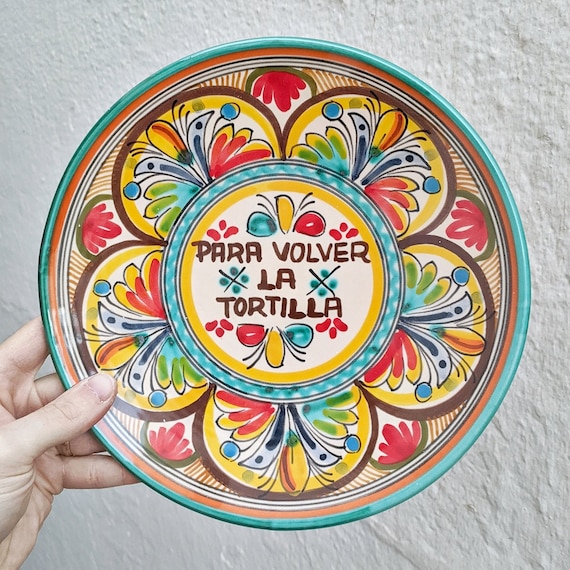A woman's hand on the left holds a decorative, circular plate up against a bright white stucco wall in the daylight. The plate has a detailed and colorful design, beginning with a turquoise border at the edges. Inside the turquoise border, there is a layer of orange, followed by black and white lines. In the center, a large blue-highlighted circle encloses another yellow circle which features a design of little red flowery dots, blue and yellow petals, and additional red flower petals positioned at the top and bottom. The phrase "Para Volver La Tortilla" is painted in brown letters within this central circle. Surrounding this core design, there are arches or semicircles that mimic the shape of a flower, further decorated with colorful elements in green, red, yellow, orange, and blue, giving the plate a festive appearance.